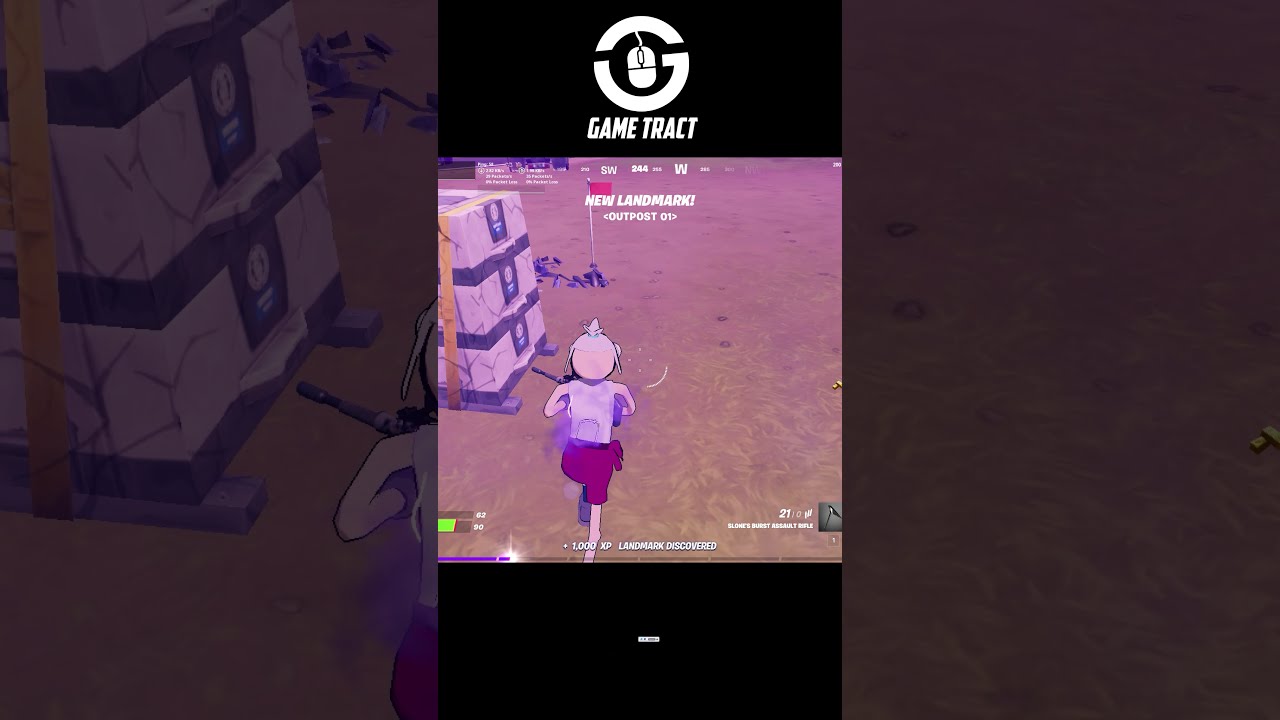The image showcases a video game screenshot presented in portrait mode with letterbox bars on the top and bottom, adding a cinematic feel. Central to the image is a character positioned on a pink-tinged open field, running left. The character is distinctive, with a pink head crowned by pointed white hair, a white shirt, and dark purple shorts revealing thin white legs. They appear to be pursued by purple spray paint and hold a machine gun with the barrel pointing left. 

To the left of the character, there are three sizable boxes, each delineated by grey lines and staggered with black tape. The front of the boxes features a dark vertical rectangle with a golden emblem in the middle. Above the character, white text reads "New Landmark Outpost 07."

The topmost section of the image displays a white circular emblem with a letter "G" and a computer mouse in the center, the mouse's cord arching upwards. Beneath the emblem, the text "game tracked" is seen. The image is flanked on both sides by larger, rectangular boxes showcasing zoomed-in sections of the main game screen, although they are dark and dimmed, adding to the ethereal and immersive atmosphere.